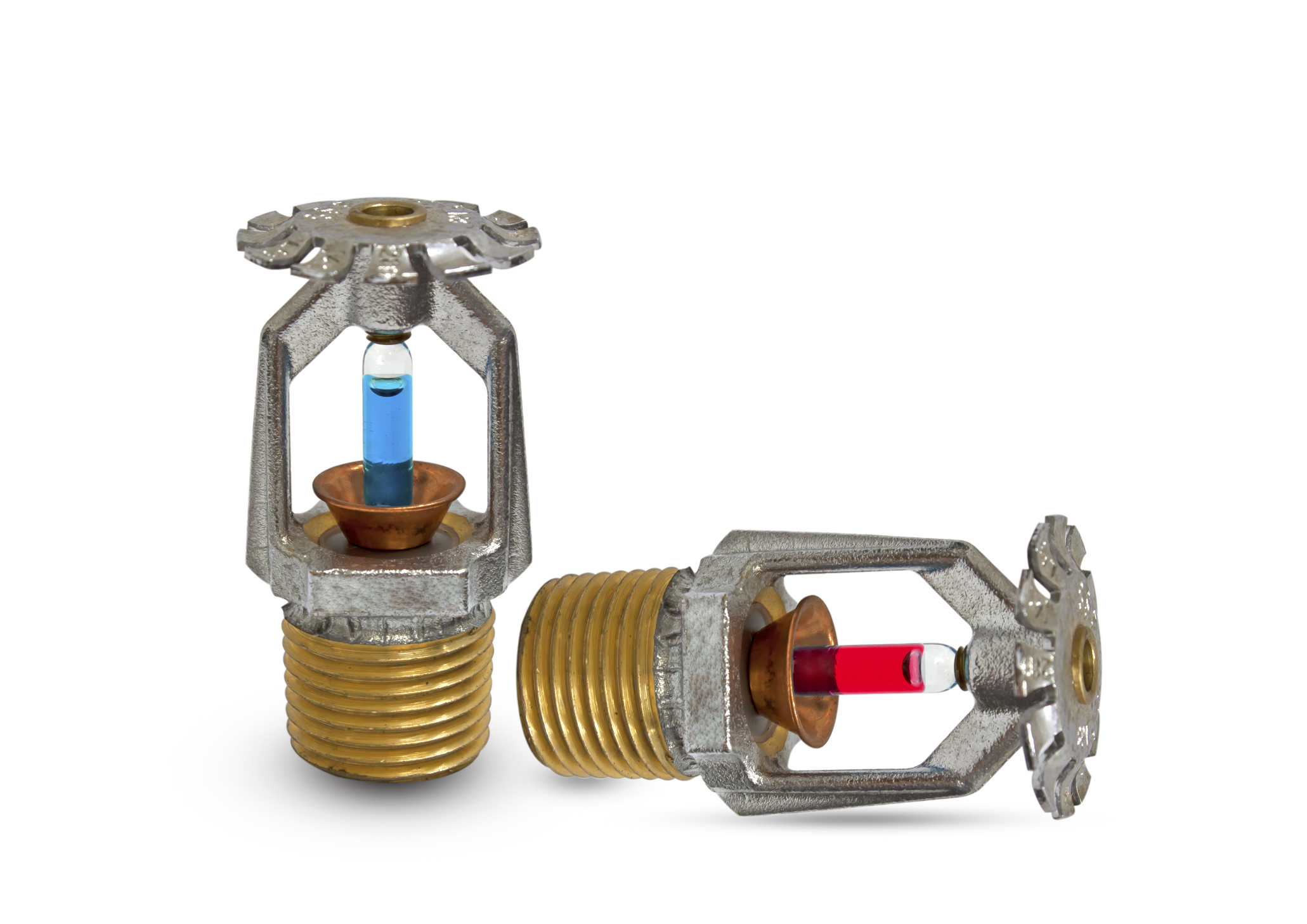The image depicts two metal sprinkler heads against a white background. Each sprinkler head has a silver, umbrella-like top, and they appear to be part of some mechanical apparatus that can be screwed in, as suggested by the gold screw threads at the bottom. At the center of the sprinkler heads, there's a bronze dish with a clear glass vial extending upwards. The left sprinkler head stands upright and contains a blue fluid almost filling the vial, while the right sprinkler head, which is lying on its side, holds a red fluid in its vial. Both vials seem integral to the function of the sprinkler heads, possibly for delivering the contained fluids into a larger system.